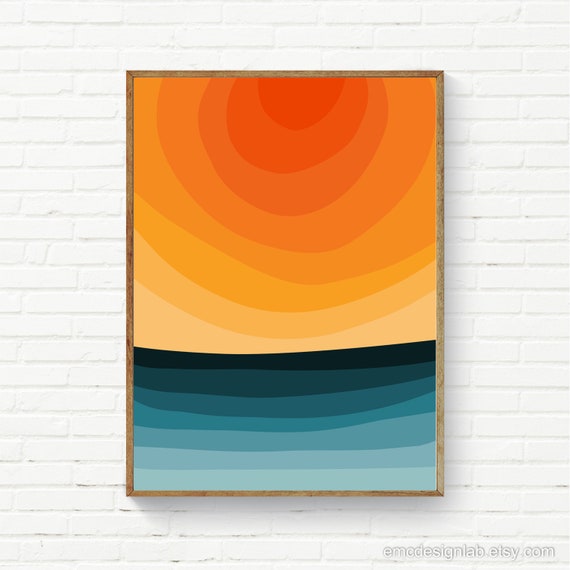A professionally shot, full-color photograph showcases a painting within a thin, brown wooden frame, mounted on a white brick wall. The painting features a minimalist representation of the sun and a body of water, divided into distinct sections of colors and shapes. At the top, concentric, incomplete half-circles start with a dark red center, transitioning through orange, yellow, and finally cream, evoking the sun. Below, straight horizontal strips symbolize water, transitioning from dark blue at the horizon to very light blue at the bottom. In the bottom right corner of the image, the watermark "emcdesignlab.etsy.com" is clearly visible. The overall composition, with its vibrant yet simplistic elements, conveys the serene interplay of sunlight over a tranquil sea.